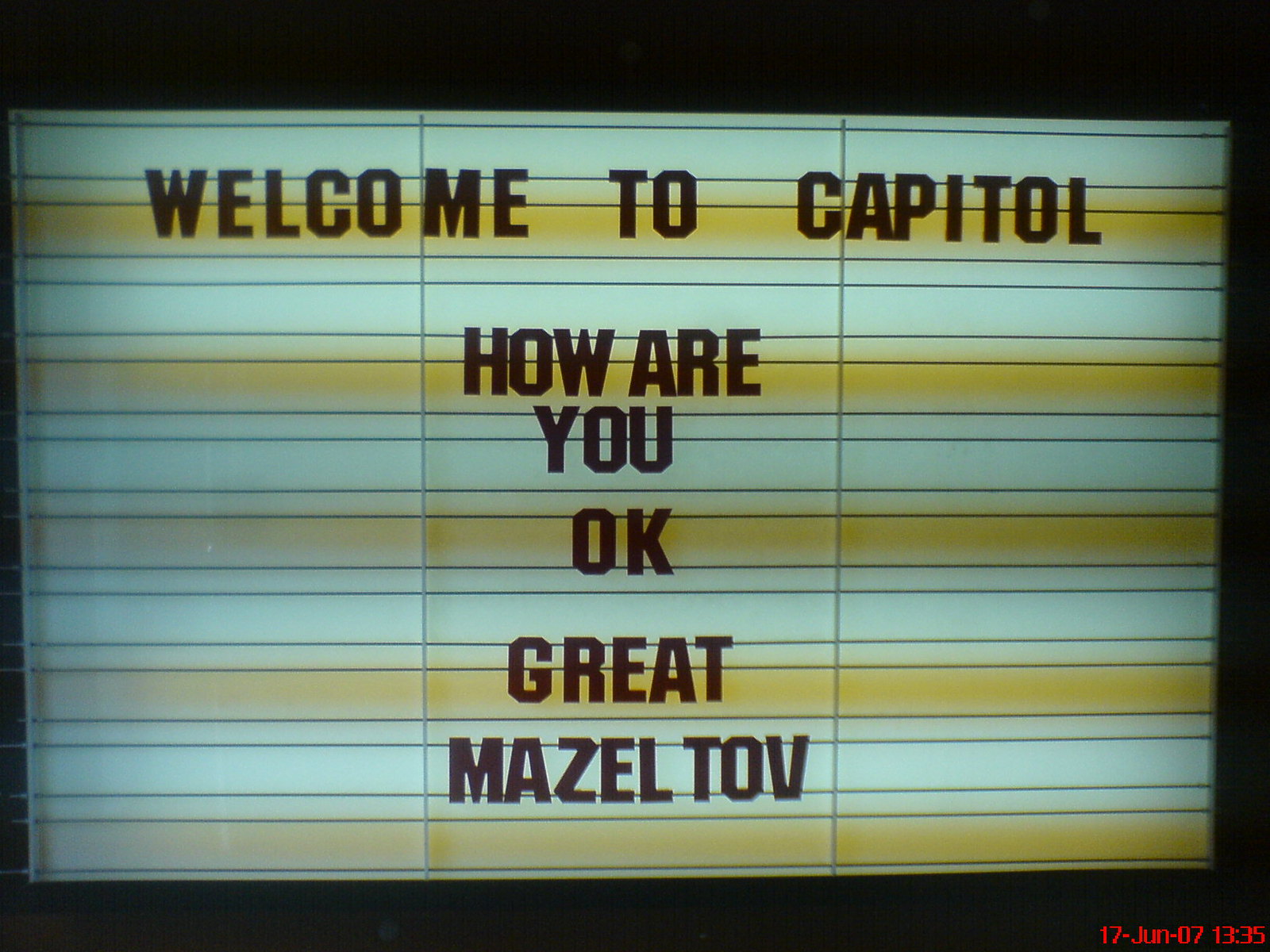The image depicts a changeable letter signboard with a dark black background and alternating white and light lemon-yellow horizontal rows. The sign features black, attachable letters spelling out the message: "Welcome to Capitol. How are you? Okay. Great. Mazel Tov." The letters are evenly spaced across the multiple rows of the sign. At the bottom right corner, small red characters indicate the date and time: "17 June 2017 at 13:35." This format and the use of the 24-hour clock suggest a European setting. The surroundings in the image appear dark, giving the impression that the sign is either illuminated at night or displayed in a dimly lit area.